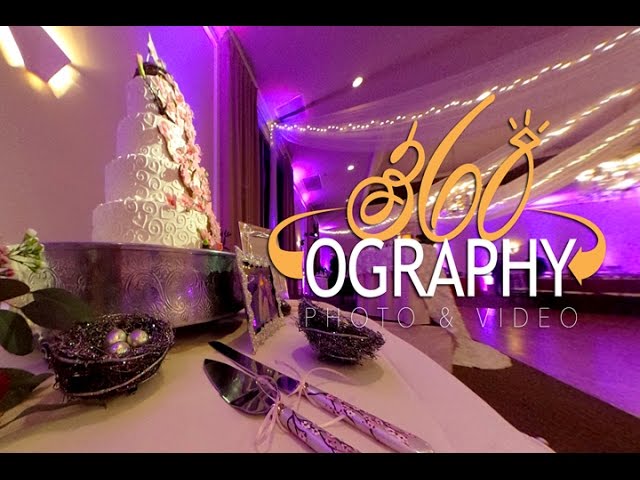This image appears to be an advertisement set in an elegant wedding venue. Dominating the foreground is a pristine, long white table adorned with an elaborate wedding cake, which is presented on a decorative platter. In front of the cake, a knife and a cake slicer are meticulously placed, indicating readiness for the ceremonial cutting. The ambiance of the scene is further enhanced by a vibrant, neon purple dance floor illuminated in the background, with twinkling white lights elegantly draped across the ceiling.

Behind the cake table, there is what seems to be a table designated for the wedding party, covered in delicate white lace. Although no individuals are present in the image, a silver-framed photograph on the wedding party table likely features the bride and groom, though it remains indistinct. Dominating the upper portion of the scene, large text in a striking combination of yellow and white reads "360ography Photo and Video," punctuating the image and highlighting the service being advertised.